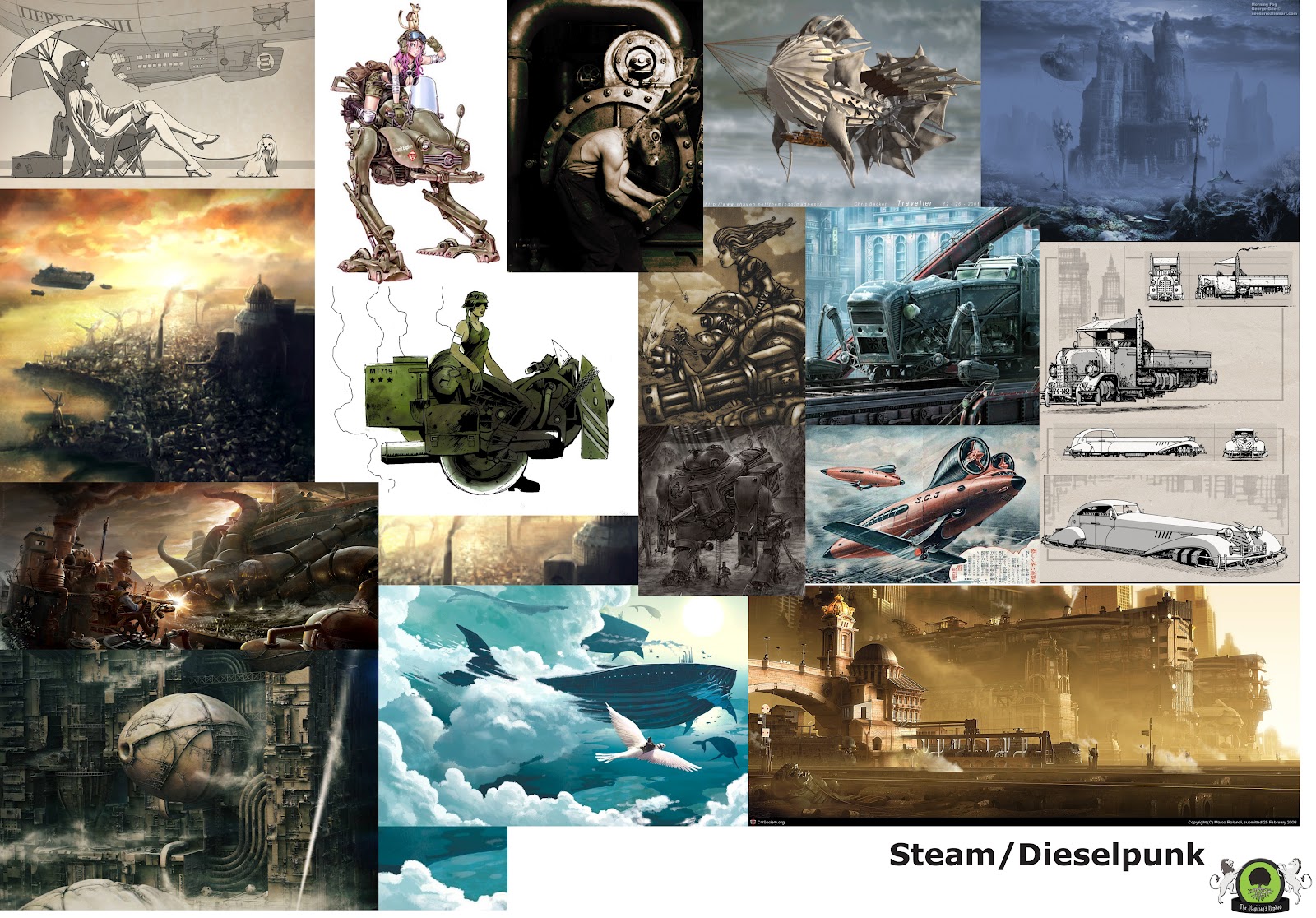This image is a digital collage consisting of multiple rectangular illustrations in various sizes and orientations, including both landscape and portrait formats. The artwork features a muted color palette with shades of gray, brown, muted blue, and muted green, giving it a subdued and somewhat dreary feel. The illustrations, which are all digital and include elements of clip art, depict a steampunk and dieselpunk aesthetic, as indicated by the black text on a white box at the bottom right of the image that reads "Steam / Dieselpunk" alongside a logo.

The central theme revolves around a dystopian, futuristic Victorian setting. The images predominantly showcase vehicles such as cars, aircraft, and boats, including one boat that intriguingly resembles a whale and another ship floating in the sky surrounded by birds. Among the various scenes, there is a large castle-like structure, a factory, and figures actively engaged with machinery—either building, working on, or using it. Notably, one image captures a woman relaxing under a sun umbrella with a dog on a leash, while a blimp hovers overhead.

Overall, the collage presents a bleak, industrial vision of the future, emphasized by dark, overcast skies and the predominance of sepia tones, black and white hues, and dark blues, reinforcing the dystopian atmosphere.